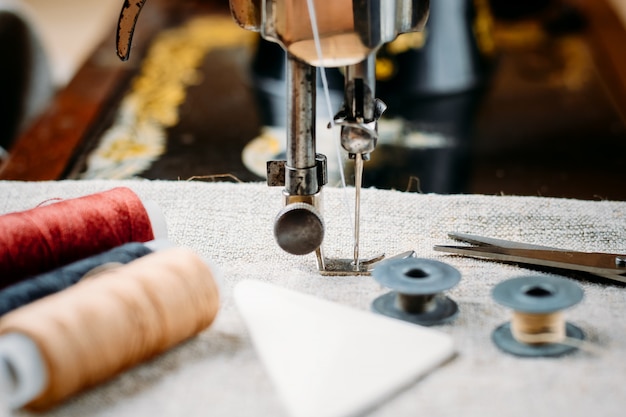In this detailed close-up photograph, the focal point is the sewing needle of a sewing machine, threaded with white thread, piercing through gray linen fabric. The sewing foot, adorned with a patina that lends it an antique appearance, dominates the center of the composition. Near the right base of the needle, the sharp part of a pair of scissors extends off-frame, also in sharp focus, while the handles remain outside the shot.

The blurred foreground features a variety of spools of thread: vibrant red, deep navy or black, and taupe or beige are discernible, along with smaller spools of darker colors and another beige spool. One spool in the center appears empty. The background, rendered indistinct due to a dramatic depth of field effect, hints at more thread colors and a dark surface, possibly wooden. The overall scene exudes an old-timey, artistic vibe, tightly focusing on the intricate action of the sewing needle amidst a blur of surrounding details.